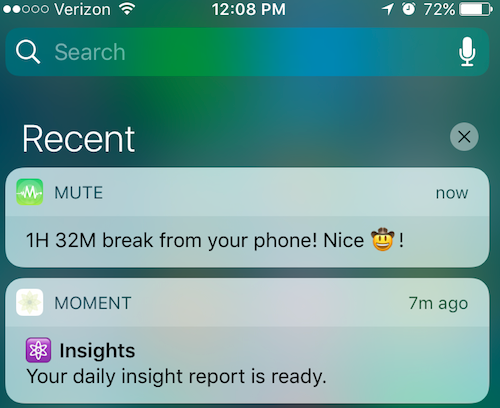This image is a screenshot of a smartphone interface, displaying both the status bar and notifications. Starting from the top right, there's a horizontal battery icon that is nearly full, depicted in white, accompanied by the text "72%". To its left, an alarm clock icon is present, along with an arrow pointing to the top right corner. Centrally, the time is displayed as 12:08 PM. On the top left, a set of five circles is visible, with two of them filled in white, followed by the carrier name "Verizon" and a fully filled Wi-Fi signal icon. 

Below the status bar, there is a search field, which is currently empty. The word "Search" and a magnifying glass icon in white are on the left side of this bracket, while a white microphone icon adorns the far right. Under this, the interface shows the section title "Recent", followed by two highlighted boxes. The first box, labeled "Mute", indicates a break from phone usage lasting "1 hour, 32 minutes" with the comment "Nice." The second box, labeled "Moment", displays further insights.

This detailed snapshot captures the user's notifications, showing various icons, connectivity status, and a focus on recent phone activity.